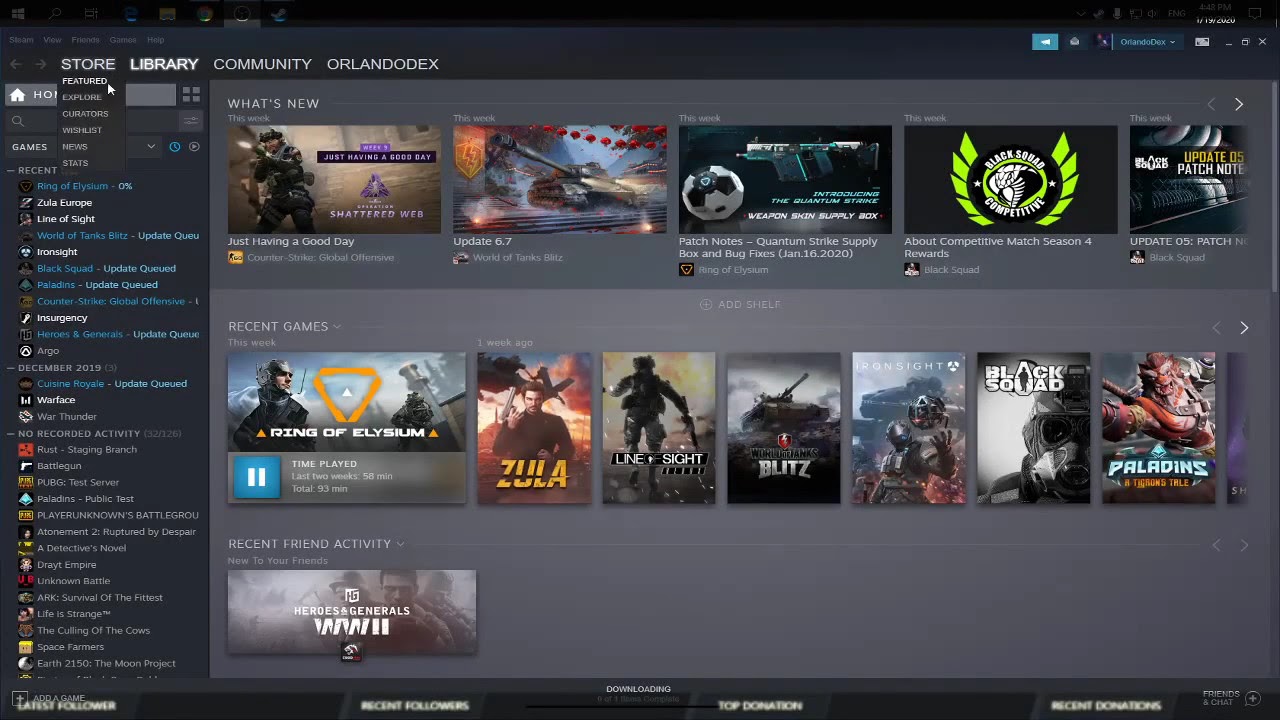This image captures a detailed view of the interface of a video game store on a digital platform. Along the top edge, there's a half-inch black border, transitioning into a two-inch dark gray band running down the left side and across the top. Below this, the background shifts to light gray. 

In the upper left corner, there are seven clickable icons designed to help users navigate the store. On the upper right side, the display shows the current time (4:48 PM), the date (January 19, 2022), the language setting (ENG), a sound icon, and a couple of other icons.

Running vertically along the left side of the interface, there are five tabs in light gray labeled "Themes," "Views," "Friends," "Games," and "Help." Beneath these tabs, arrows pointing left and right are visible, and below these, sections labeled "STORE," "LIBRARY," and "COMMUNITY" are prominently displayed in uppercase letters. The "STORE" section is highlighted.

The interface also includes a dropdown menu under "Our Orlando DX Store," which provides options such as "Featured," "Explore," "Curators," "Wishlist," "News," and "Stats," all in white text. A cursor arrow points towards the "Featured" section, indicating user interaction.

The left panel of the interface shows conversations among users discussing various games. This runs down the left side of the screen. 

In the main section to the right of this panel, under a header labeled "What's New" in all capital white letters, there is a horizontal line extending across the screen, with a gray greater-than symbol pointing left and a white greater-than symbol pointing right. Below this header, the section titled "This Week" displays five games (four fully visible and one partially cut off), with their names and additional information provided.

Further down, a gray bar labeled "Recent Games" leads into another section titled "This Week," showcasing one large square game icon followed by six rectangular game icons. 

The bottom part of the interface features a section labeled "Recent Friend Activity," with the game "Heroes and Generals: World War II" mentioned.

This comprehensive layout offers a detailed snapshot of the video game store's user interface, highlighting various navigation elements and current content offerings.